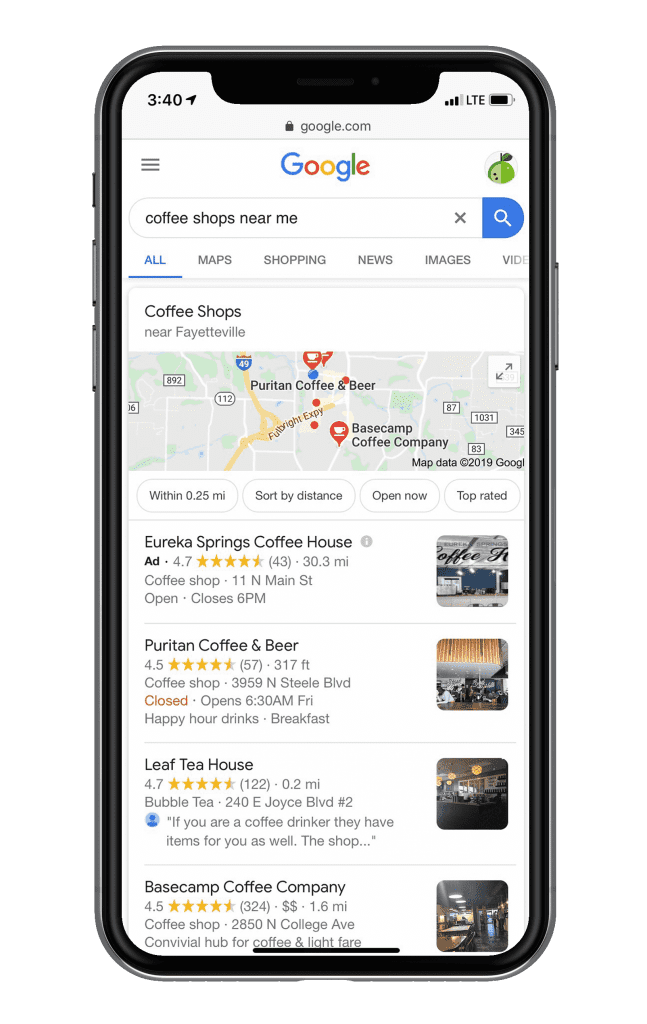The image depicts a cell phone screen displaying a search for coffee shops. At the top of the screen, the time is 3:40, and the battery is almost fully charged, with three bars of Wi-Fi connectivity. The screen is on the Google search engine, where the query "coffee shops near me" has been entered. 

The search results are focused on coffee shops in Fayetteville. A map displays various coffee shop locations, with two notable markers highlighted. Below the map, there is a list of four coffee shops. The first result is "Eureka Springs Coffee House," which features an advertisement and boasts a rating of 4.7 stars. The second result is "Puritan Coffee and Beer," which has a slightly lower rating of 4.5 stars and is located just 317 feet away from the user. In contrast, Eureka Springs Coffee House is 30.3 miles away, indicating that the results are not filtered by proximity.